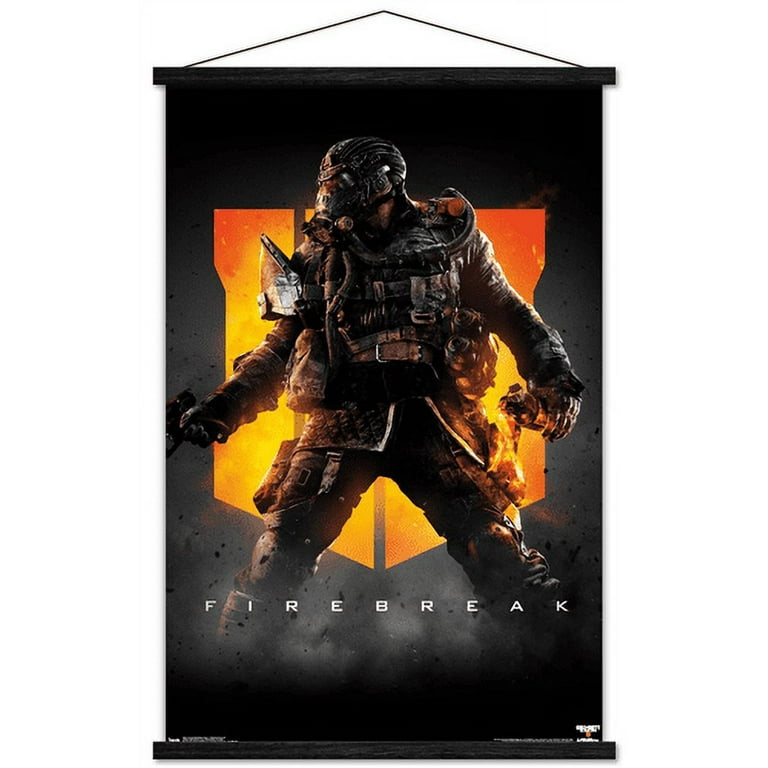The image features a scroll poster held in place by wooden rods at the top and bottom and hangs from a string. The poster itself has black borders with a dramatic, fiery background in shades of bright orange and yellow, suggestive of intense flames. At the center stands a figure, ambiguously human, dressed in elaborate, military-style gear. The figure is fully armored with thick protective clothing, including a heavy vest adorned with various straps and pockets, high boots, and a tight black helmet with a gas mask that entirely conceals the face. The stance is wide-legged, with the right hand gripping what appears to be a gun and the left hand holding an indistinct object that might be a grenade or flashbang. At the level of the shins, the words "FIRE BREAK" are prominently displayed in white letters. Additionally, there seems to be smaller, unreadable text in both lower corners.